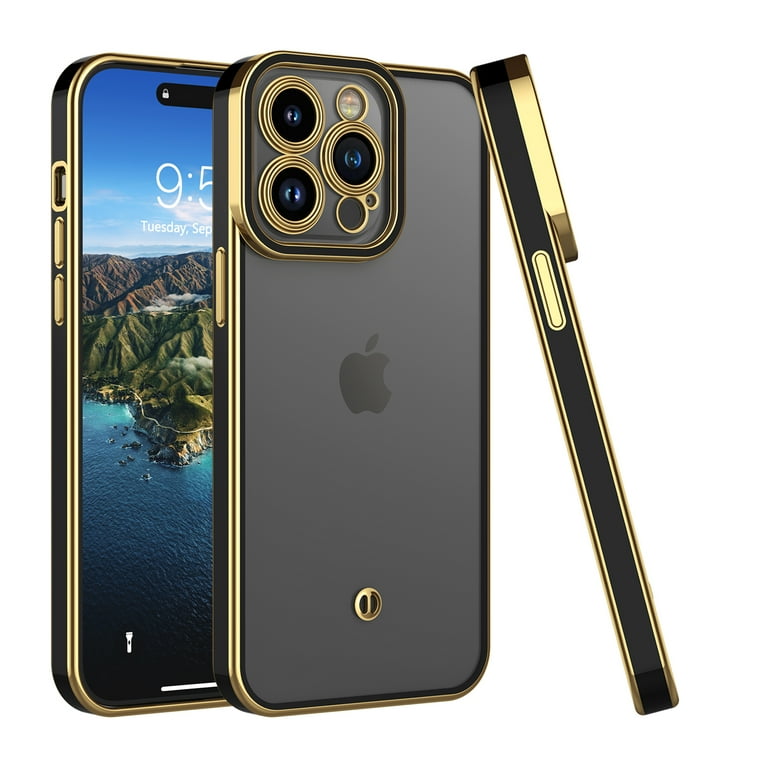The image showcases three distinct views of a sleek, space gray Apple iPhone model, possibly a concept design for a future release. The phone is encased in a stylish black and gold frame. The primary back view reveals a sophisticated triple-lens camera setup in the top corner, each lens adorned with a gold outline, and the iconic Apple logo centered on the dark gray surface. To the right, a slim side profile highlights a gold-trimmed black power button, emphasizing the phone's elegant design. Behind the main phone image, a partially covered front view displays the lock screen, featuring the time as 9:50-something on a Tuesday in September, with a vivid image of an island amidst a bright blue ocean. This screen layout hints at advanced features like the flashlight icon and a dynamic island at the top, which could indicate features beyond the iPhone 14 series.